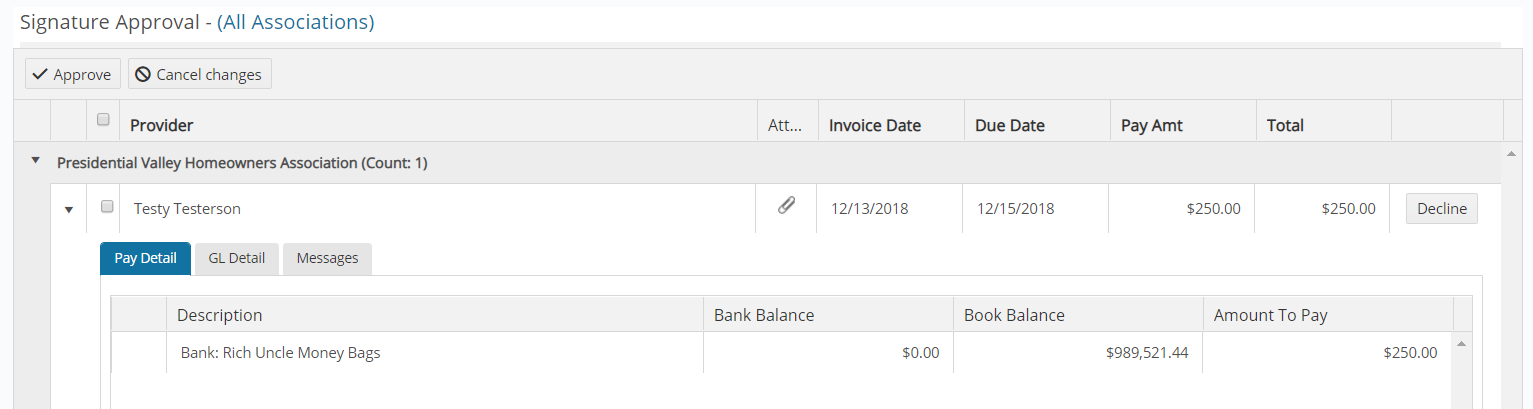The image depicts an invoicing software interface, predominantly colored in shades of gray, black, and white. At the top, the title bar reads "Signature Approval – All Associations". Beneath this, buttons for "Approve" and "Cancel Changes" are prominently displayed. The main section features columns labeled "Provider," "Invoice Date," "Due Date," "Pay Amount," and "Total."

The table within this section lists one entry for the "Presidential Valley Homeowners Association." The provider is noted as "Testy Esterson," indicating that this may be a test entry. The invoice date is December 13, 2018, with a due date of December 15, 2018. The entry shows a pay amount and total of $250, with a "Decline" button available for action.

Below the table, there are tabs labeled "Pay Detail," "GL Detail," and "Messages." Inside the "Pay Detail" tab, the description mentions "Bank: Rich Uncle Moneybags" with a bank balance of zero but a book balance exceeding $989,000. The amount to be paid is listed as $250. The program appears to be in a testing phase, likely to evaluate its functionalities and user interface. The overall design is minimalistic and utilitarian, without any vibrant colors.